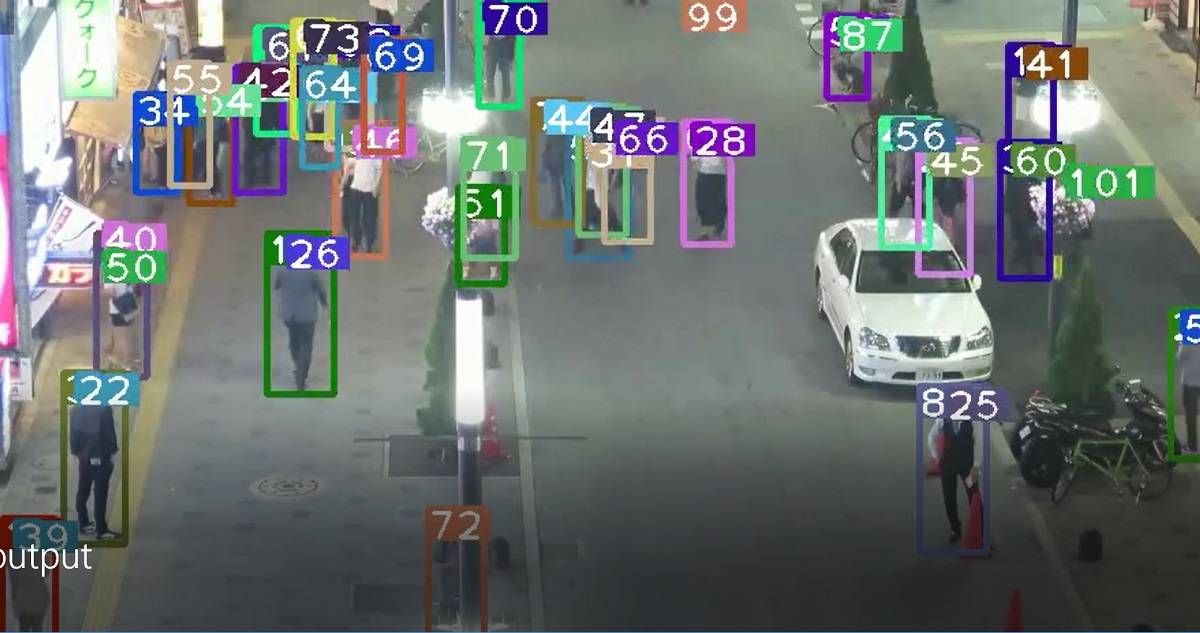A security camera screenshot captures a bustling street scene. On the left side of the image, the edges of several buildings are visible, adorned with various fluorescent-lit signs. These signs, featuring white and black lettering in an Asian script, provide a vibrant array of advertisements against the cityscape. The street itself is a wide, brick-paved sidewalk that transitions into a black asphalt road. 

A white car is parked on the right side, while numerous pedestrians fill the scene, walking in various directions. The people, dressed in a mix of casual attire in colors such as white, black, gray, blue, and green, are marked by colored squares overlaid on the image. These squares, in hues of green, blue, and light green, each contain a number in white text, ranging from 28 to 101. 

The numerical annotations suggest a form of tracking or identification, potentially counting the number of people or possibly indicating another type of data such as a social credit score, common in certain areas like China. The presence of these markers adds a layer of digital analysis to the otherwise everyday urban environment.